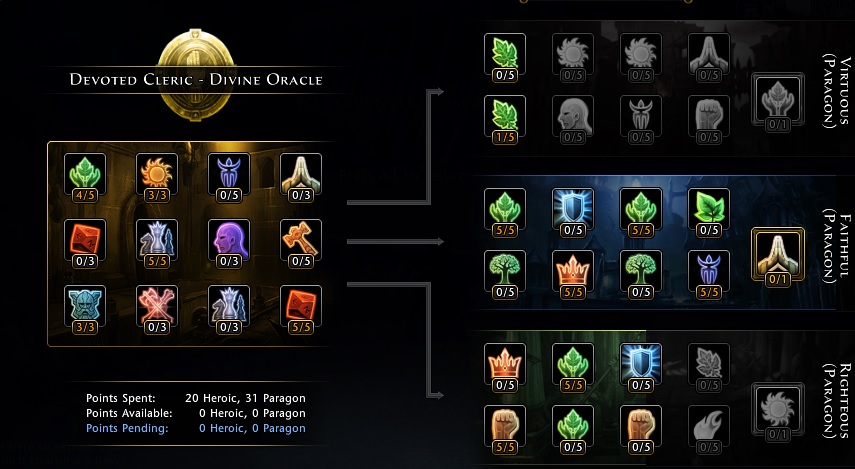The image is a horizontally aligned rectangular screen with a solid black background that resembles a character progression menu from a fantasy video game. In the upper left-hand corner, there's a gold oval-shaped medallion with the text "Devoted Cleric - Divine Oracle" over it. Below this, there is a 4 by 3 grid of 12 bright, colorful icons, each accompanied by numerical values indicating points (e.g., a green flower icon labeled "4/5" in orange). Under this grid, there's a table detailing points management which includes "Points Spent: 20 Heroic, 31 Paragon; Points Available: 0 Heroic, 0 Paragon; Points Pending: 0 Heroic, 0 Paragon."

To the right of this section, the screen depicts three vertically aligned categories of more icons, each classified under different headings: "Virtuous Paragon," "Faithful Paragon," and "Righteous Paragon." Each category displays several icons with some lit up and others grayed out, indicating different statuses or levels of achievement within the game. The top section ("Virtuous Paragon") features icons, including two green leaf symbols with "0/5" and "1/5." The middle section ("Faithful Paragon") and the bottom section ("Righteous Paragon") similarly have clusters of lit and unlit icons, reflecting different stages of character abilities or stats within the game's character progression system. The overall design conveys a space-age, mystical gaming interface.